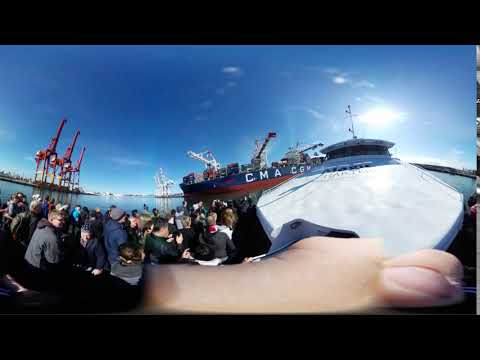The image captures a bustling seaport scene under a vivid blue sky, dotted with a few clouds and the distorted sun. In the foreground, 20 to 40 people clad in jackets and hats, suggesting cooler weather, stand on the shore, gazing toward the activity in the harbor. To the left, there's a trio of red cranes towering over the scene, poised to load or unload ocean-going vessels. Dominating the center is a blue and red cargo ship labeled "C.M.A," its deck and the sign partially obscured but still visible. The ship, industrial and imposing, is docked, possibly being loaded or unloaded. The scene has a surreal, almost virtual reality quality, with shapes and details blending in a slightly disorienting way. Overall, the detailed tableau depicts a heavily industrialized port area, its waterfront bustling with machinery and human activity, extending off into the distant city skyline.